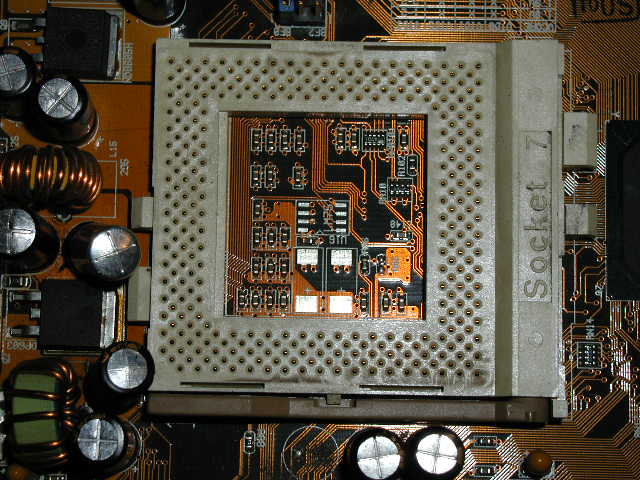The image showcases a detailed close-up of an older model motherboard, characterized by a rich mix of copper, black, silver, and rusted orange hues. Along the bottom and left side, a series of capacitors wrapped in black plastic with silver tops marked by X's are visible. A prominent copper coil sits about a third of the way down on the left, flanked by condensers and box-shaped black objects, possibly transformers. The motherboard is adorned with intricate white circuit lines, especially concentrated on the bottom right and top right sides.

Dominating the center is a metal square socket labeled "Socket 7," which features multiple holes and reveals underlying circuitry through a central cutout. This socket is intended for seating a CPU, integrating it into the motherboard. Additionally, there are several large silver knobs, with counts reaching up to eight, complemented by smaller brown and larger green knobs. The overall layout includes multiple other capacitors and printed circuitry patterns intricately woven throughout the board, making this a highly detailed and complex electronic component.